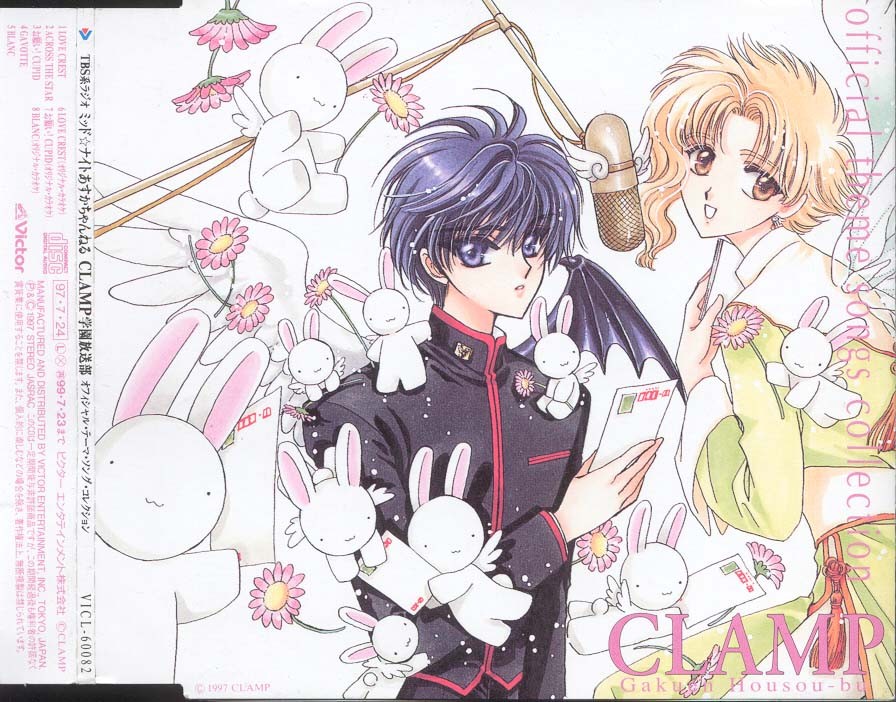The album cover for a music album features an intricate anime-style illustration. At the center, a man with purple hair and a black high-collar coat with red trim is depicted alongside a woman with blonde hair in a green dress with white sleeves and a sash. Both characters face a gold microphone adorned with wings on either side. The man has contrasting black and white wings behind him, symbolizing duality, while the woman also appears to have white wings. Surrounding them, various stylized cartoon rabbits with angel wings are scattered throughout the scene, along with an array of flowers. An inscription along the right side reads "Official Theme Songs Collection" in vertical text. In the bottom right corner, in pink text, the caption reads "Clamp Gakuin Hoso B." The overall image is vibrant and detailed, offering a whimsical yet elaborate visual experience.